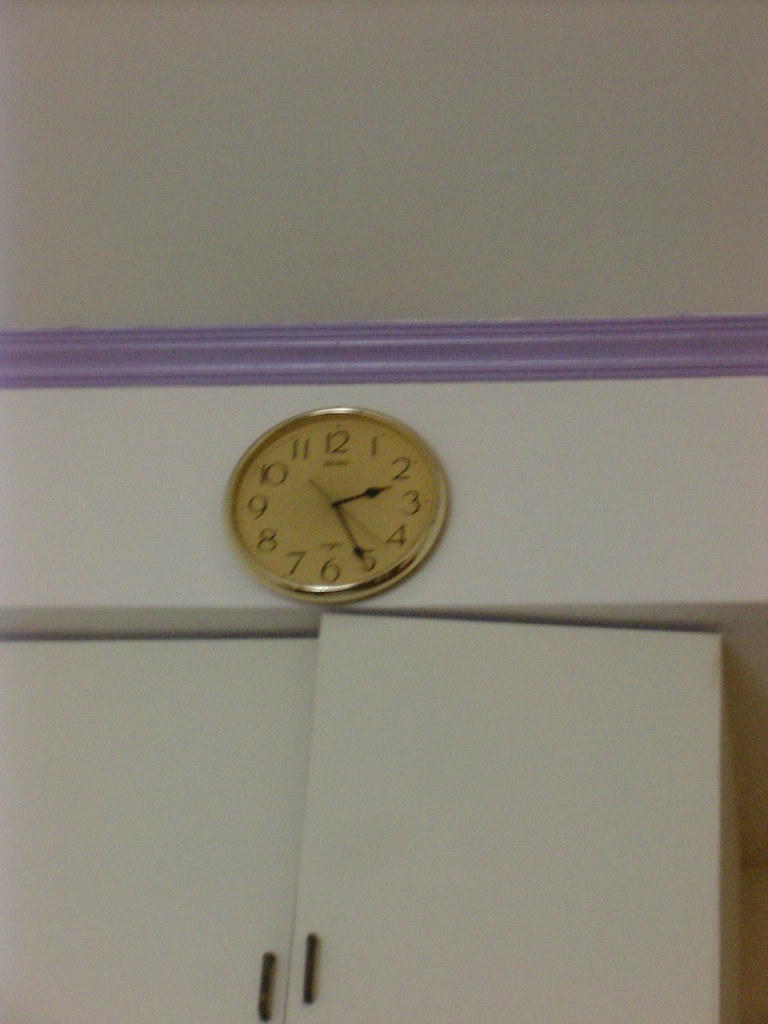The image captures a vintage-looking wall clock positioned just a fraction below the ceiling. The clock's light brown background contrasts elegantly with its gold bezel, adding a touch of classic charm. It's almost touching the upper edge of a two-door cabinet, barely clearing the bezel, emphasizing its slightly off-center mounting. The cabinet itself is pristine white with vertical brown handles, suggesting a modern yet subtle design. The surrounding environment features an off-white wall, a light gray ceiling, and blue-gray trim where the ceiling meets the wall, complementing the clock’s vintage aesthetic. This thoughtful arrangement highlights the clock's intricate details and the harmonious blend of colors in the room.